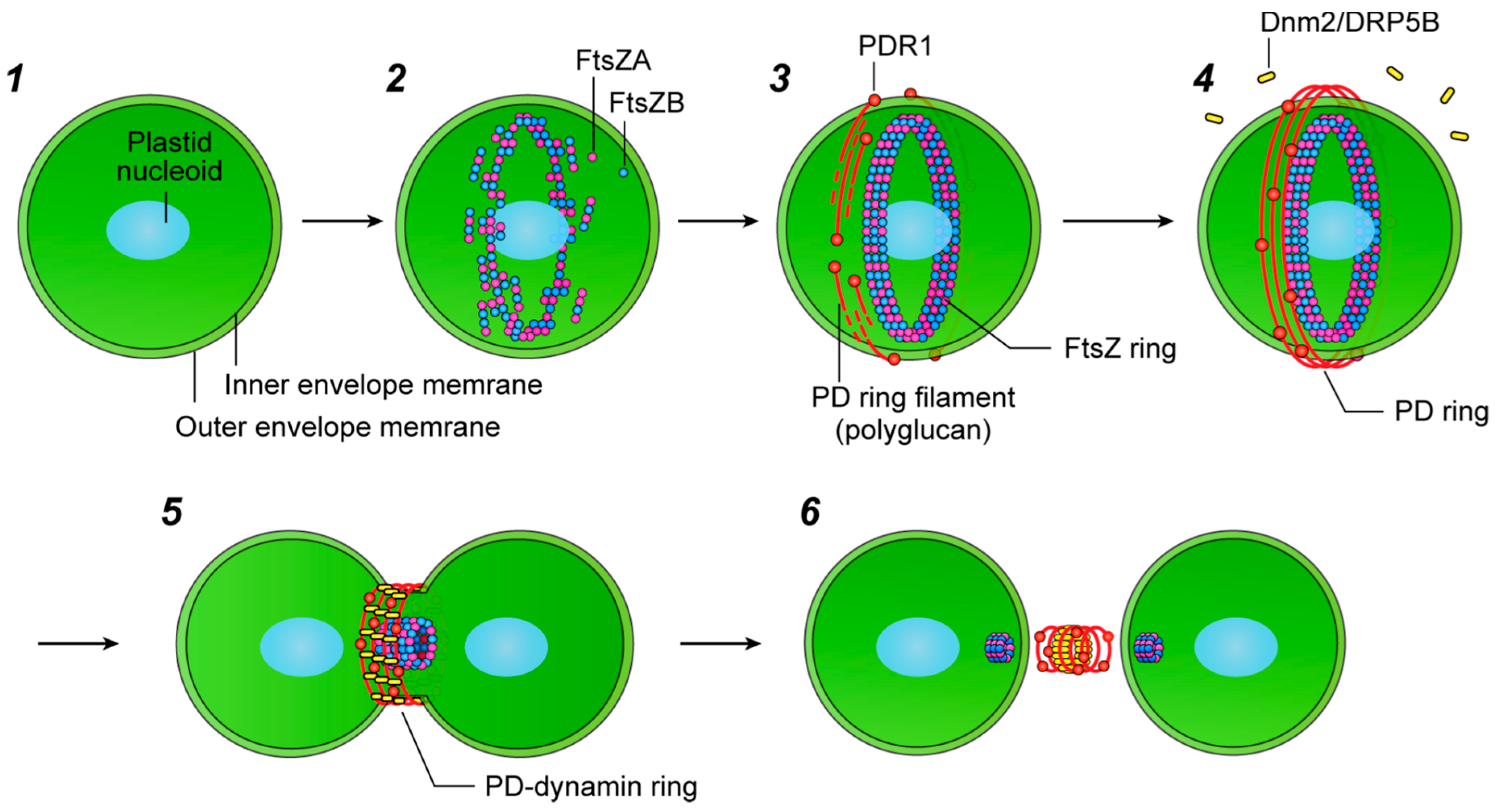This image displays a detailed biological diagram illustrating the six stages of plastid nucleoid division within cells, set against a white background. Stage 1 features a single green circle containing a blue center labeled "plastid nucleoid," along with inner and outer envelope membranes. An arrow points to Stage 2, where small pink and blue dots begin to appear around the nucleoid. In Stage 3, these dots form a ring pattern around the center, alongside red lines and dots labeled "PD ring filament polyglucan" and "PDR1" as well as "FTSZ ring." The diagram progresses to Stage 4, showing similar features with additional labeling for "PD ring DNM2-DRP5B." In Stage 5, the diagram depicts two green circles connected by the PD ring and filament structures. Finally, Stage 6 illustrates the complete division, resulting in two separate green circles, each with its ring and plastid nucleoid, signifying the end of the division process.